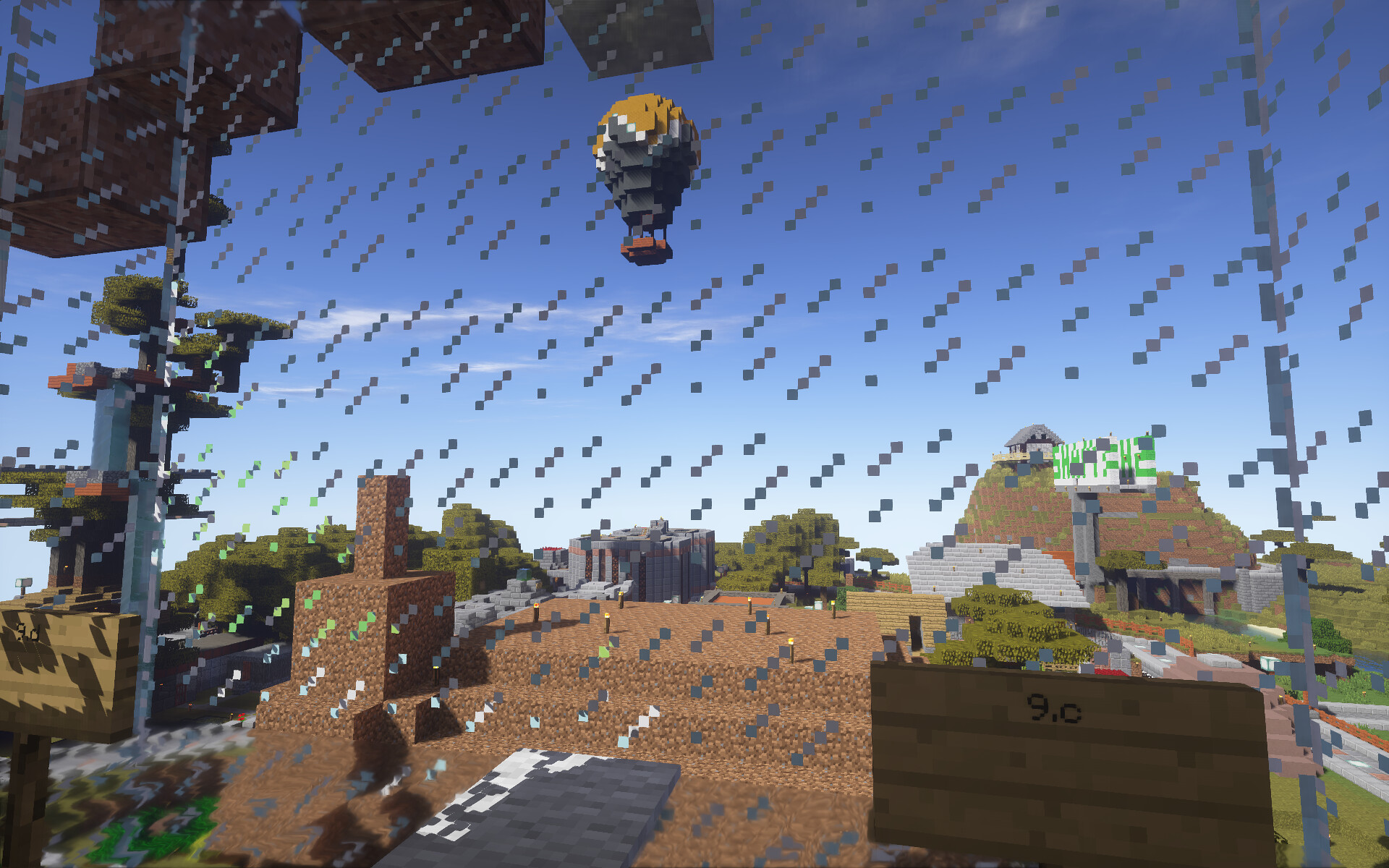This is a detailed screenshot of a video game, characterized by a distinct pixelated, computer graphic style. The image is notably filled with video distortion, featuring numerous small, diagonal, blotchy lines made of little squares that create a rain-like appearance across the scene. Dominating the upper middle of the image is a hot air balloon with a yellow top, grayish sides, and a red basket, set against a blue sky with some clouds. 

In the background, there's a tall structure that could either be a skyscraper or a tower, and towards the left, there's another block-like structure, potentially representing trees or additional skyscrapers. The lower part of the image includes a landscape with various buildings and rooftops, suggesting a suburban or cityscape view. On the right, there's a brown rectangular scoreboard or sign that reads "9.0" next to a pole. The foreground and immediate area beneath the balloon include what looks like brown stone stairs and pathways, indicating it might be part of a game level where the player could navigate. Overall, the screenshot captures a blend of urban and scenic elements through its pixelated and graphically stylized presentation.